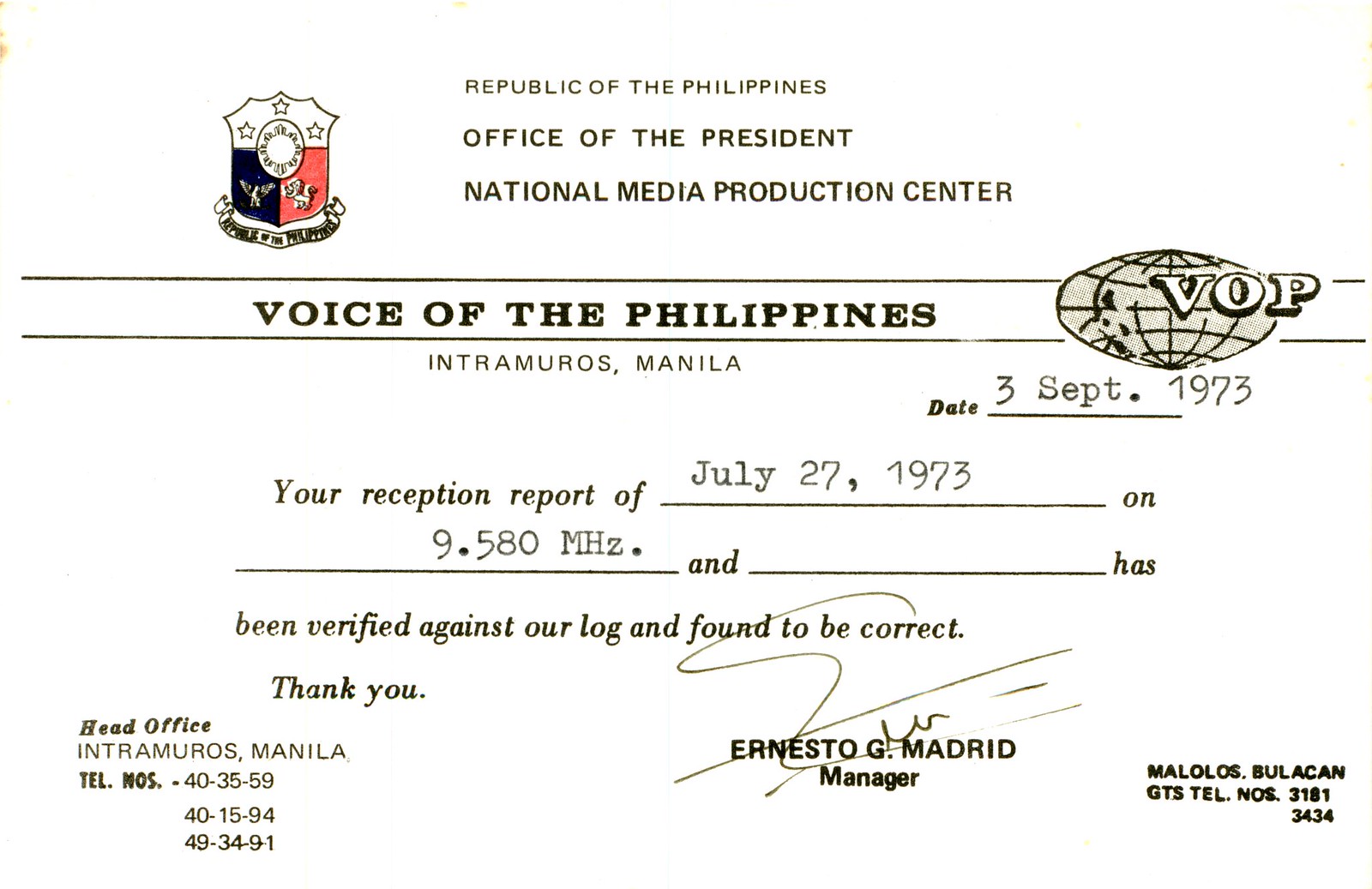This color photograph captures a verification receipt from the Republic of the Philippines, issued by the Office of the President's National Media Production Center, Voice of the Philippines. The document, occupying the entire image, features a multi-color letterhead with the Republic's coat of arms in the upper left corner. The central heading reads: Republic of the Philippines, Office of the President, National Media Production Center, Voice of the Philippines, Intramuros, Manila. Below this header, the receipt is dated September 3, 1973, verifying a reception report from July 27, 1973, on 9.580 megahertz as correct. The acknowledgment is signed by Ernesto G. Madrid, Manager, with contact details including telephone numbers 403559, 401594, 493491. The prominent colors in the image are white, black, red, yellow, and gray, framing a focused shot of this official communication.